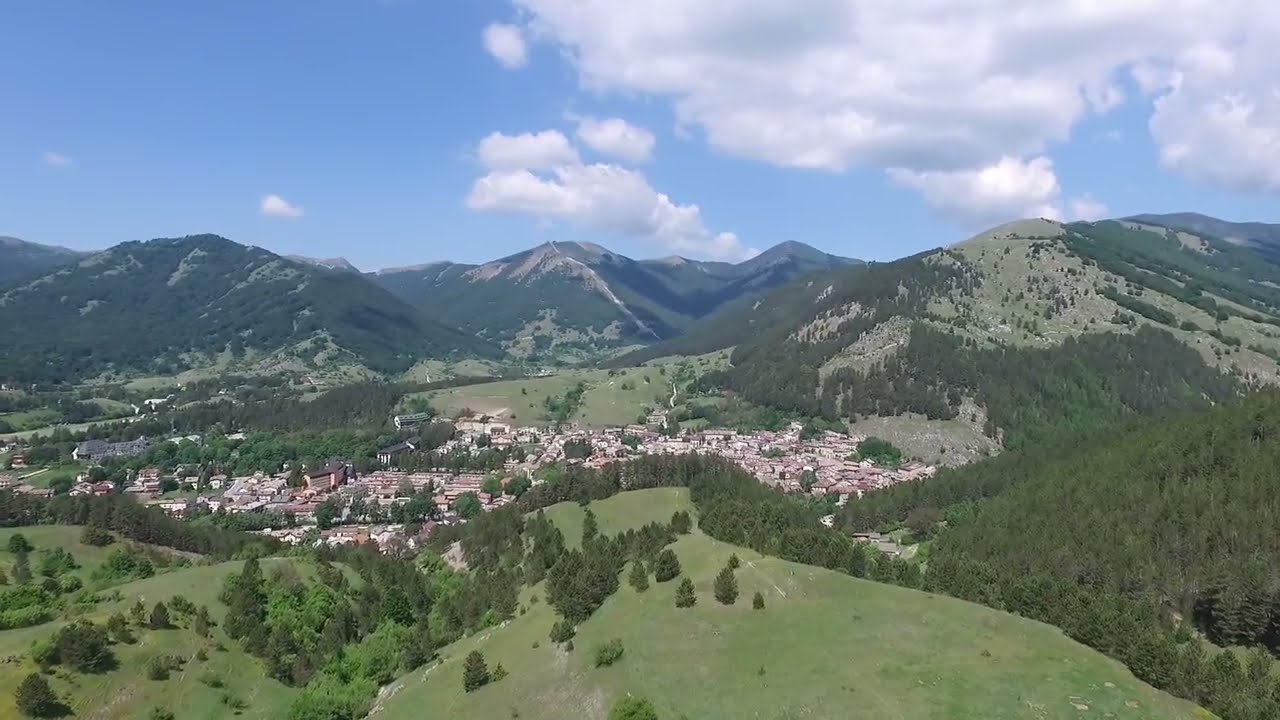The image captures a picturesque aerial view of a small town nestled in a lush mountain valley during a sunny day. The upper third of the photograph features a bright blue sky dotted with thick white clouds, particularly concentrated towards the right-hand side. Below, the expansive mountain range is blanketed with green grass and interspersed with dense patches of pine trees. This verdant landscape dips gracefully into a broad valley where the town resides.

The town itself is relatively compact, stretching approximately 15 blocks long and 4 blocks wide. It appears to be organized along a central main street, which, although not directly visible, clearly structures the alignment of closely clustered brown houses. To the bottom left and extending towards the center of the image, the town is surrounded by rolling, grassy foothills and scattered forested areas. A road can be seen winding along the foothills, disappearing into the distance. The scene is completed by grassy fields and additional clusters of trees that frame the bottom right of the image, enhancing the serene, pastoral atmosphere. 

Overall, the image beautifully encapsulates a tranquil, bucolic town enveloped by the majestic embrace of nature.